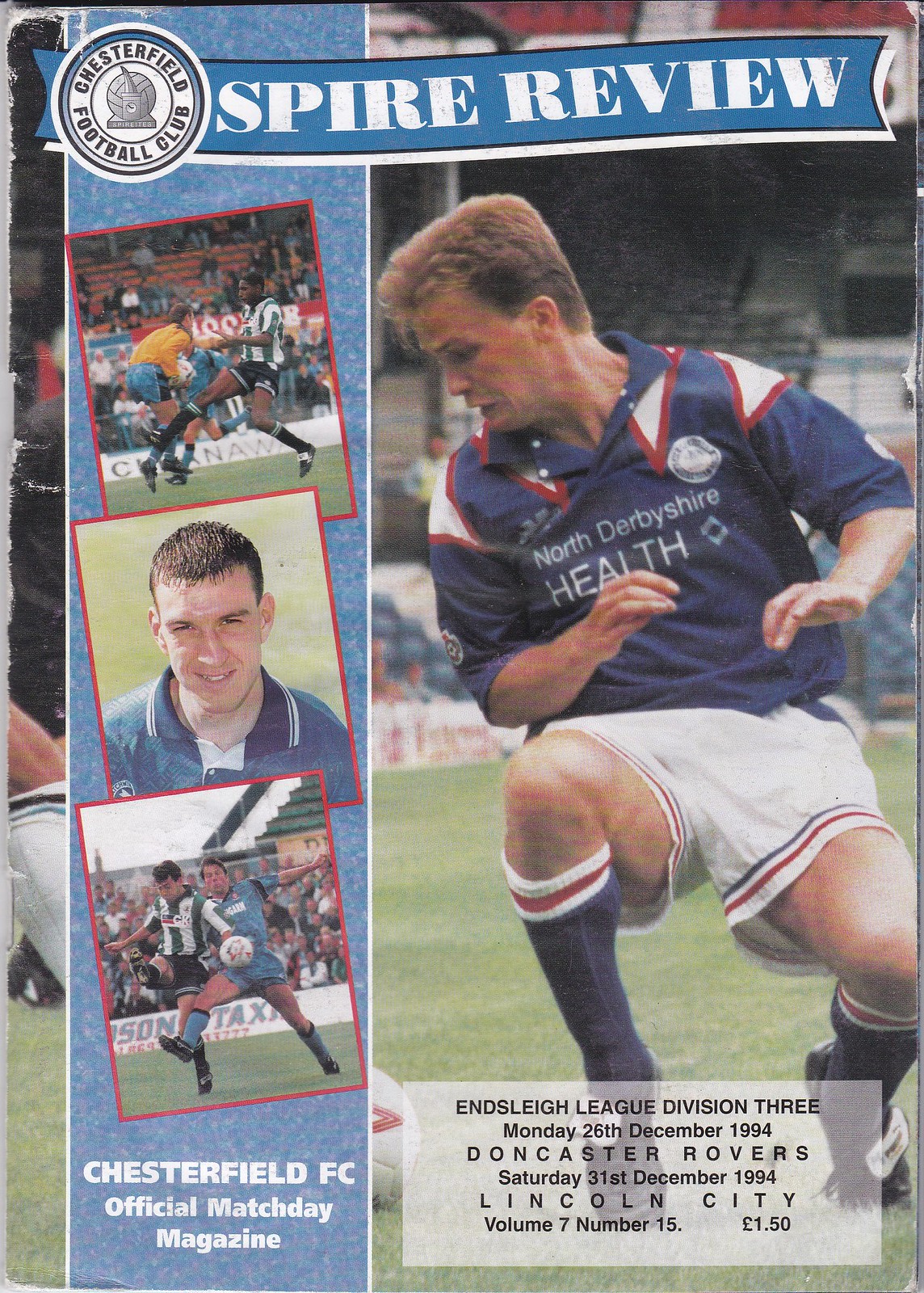This is the front cover of the official Chesterfield Football Club Match Day magazine, titled "Spire Review." Dominating the cover is a large photograph of a player from Chesterfield FC. The player is wearing a royal blue jersey with "North Derbyshire Health" printed on it, paired with white shorts and blue socks. He’s crouched down, gazing intently at a soccer ball positioned near his right foot.

On the top left of the cover, the Chesterfield Football Club logo is prominently displayed, with "Chesterfield Football Club" written next to it. To the right, the title "Spire Review" is emblazoned in white letters.

Adjacent to the player's image, there are three smaller photographs aligned vertically: the top one shows three players contesting for the ball, the middle is a close-up headshot of a player in a blue jersey, and the bottom features two players battling for control of the ball during a match.

Towards the bottom of the cover, inside a semi-transparent white rectangular box, important match details are listed in black text. It reads: "Chesterfield FC Official Match Day Magazine," followed by "Inslee League Division III," with dates and opponents listed as "Monday, 26 December 1994, Doncaster Rovers," and "Saturday, 31st December 1994, Lincoln City." It also notes "Volume 7, Number 15" and the price "£1.50."